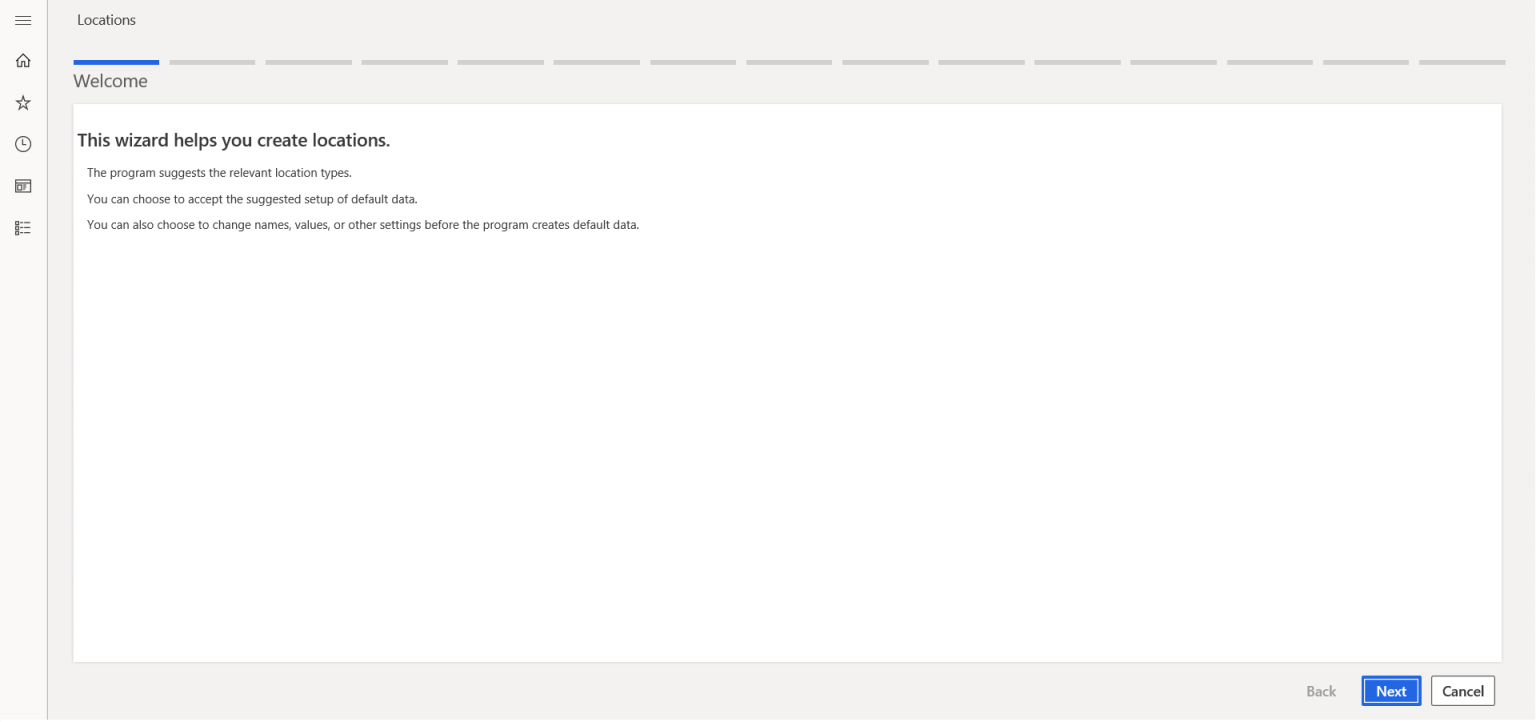A vibrant morning scene is depicted inside a modern building, adorned with star-shaped decorations and a prominent clock. The interior is warmly illuminated by a total of fifteen lights, casting a welcoming glow throughout the space. The image includes a detailed instructional text overlay, which states: "This wizard helps you create locations. The program suggests a relevant location type. You can choose to accept this or set dual tables. You can also choose to change names, values, or other settings before the program creates default data." The background of the interface is predominantly white, contributing to an uncluttered and clean aesthetic. In the bottom right corner, there is a navigation element featuring a blue square and a white square, with a black "Cancel" button centered within the latter. The scene is rich with instructional detail, clearly guiding users through the process of utilizing the location-creation wizard.